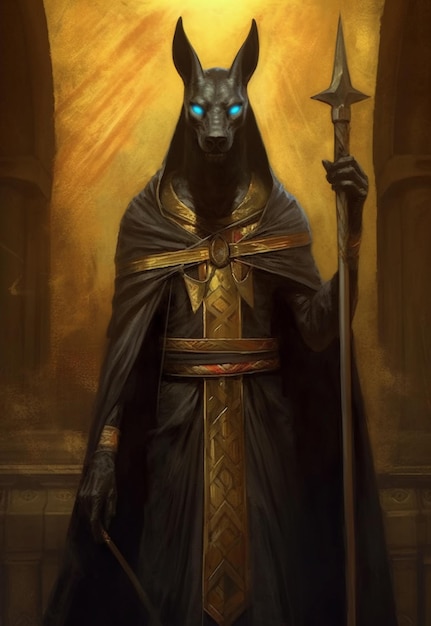This image showcases a striking drawing of a humanoid figure with a distinctly Egyptian style, paired with modern or futuristic touches. The figure features a black dog-like face with pointed ears and luminous, eerie light blue eyes that draw immediate attention. The transition from the dog-like head to a more human-like body is seamless, enhancing its mystical aura. It is adorned in a regal black and gold outfit, complete with a black cape secured by a golden belt. The ensemble extends into a long, flowing robe that contributes to its majestic presence. In its left hand, the figure grips a golden spear, while the right hand wields a knife or a stick, held down. The background boasts a textured, golden hue resembling stone or sandstone, which adds depth and a rich, ancient ambiance to the artwork.